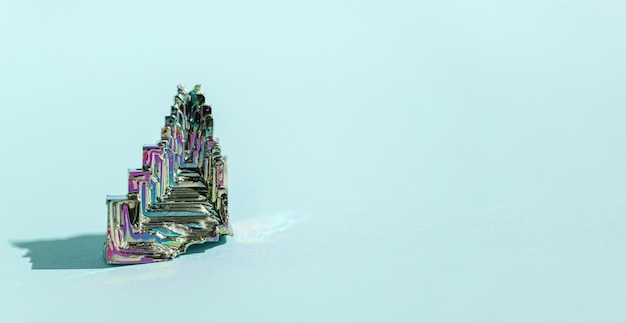The image features a light, pale blue background with a single, striking object at the center. This object is a geometric, iridescent form that vaguely resembles a nugget or a crystal, casting a shadow to its left indicating the light source is from the right. The object is highly colorful, showcasing an array of hues including silvers, blues, purples, greens, pinks, and yellows, which gives it a rainbow-like quality. It appears almost metallic or like glass with a complex, shimmering surface. The formation has an intricate, almost architectural structure that could be compared to a cityscape or stairway, with sections that seem to be broken or melted, especially at the bottom right. Its intricate, pointed top gradually squares off as it descends, somewhat resembling a pyramid, adding to its mysterious and otherworldly allure.